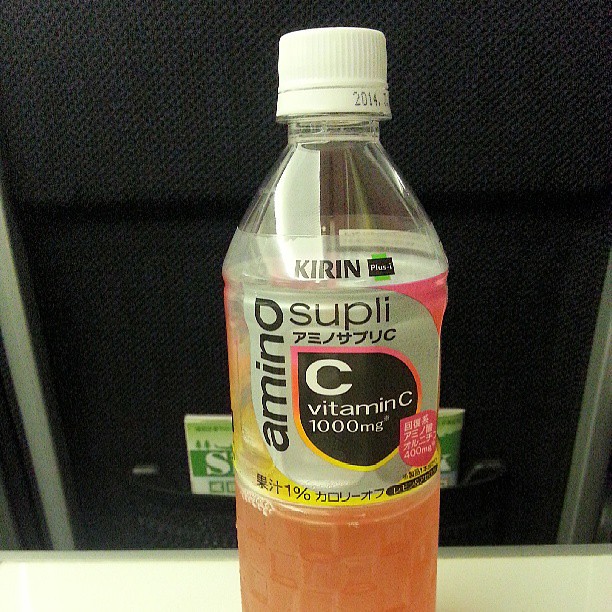This close-up photo features a partially consumed bottle of a Japanese soft drink from Kirin, famously known for Kirin beer. The clear plastic bottle, adorned with a white lid marked "2014," holds a vibrant strawberry lemonade-colored liquid at the bottom. The upper part of the bottle is transparent, showcasing a checkerboard or woven texture near the bottom. The label prominently displays "Amino Supply" (stylized as "S-U-P-L-I"), with "Amino Supply C" written in katakana, emphasizing its 1000 mg vitamin C content. A striking black teardrop shape edged in pink, yellow, and orange features a large white "C" along with a smaller pink seal adorned with white kanji. The bottle rests on a white surface with a slight lip, possibly a countertop with a low backsplash. Behind it, there seems to be a black fabric-covered piece of furniture, equipped with a sewn-on pocket containing a pamphlet in shades of light and dark green. This setting might suggest the back of a seat, likely on an airplane, given the tray-like appearance of the surface.